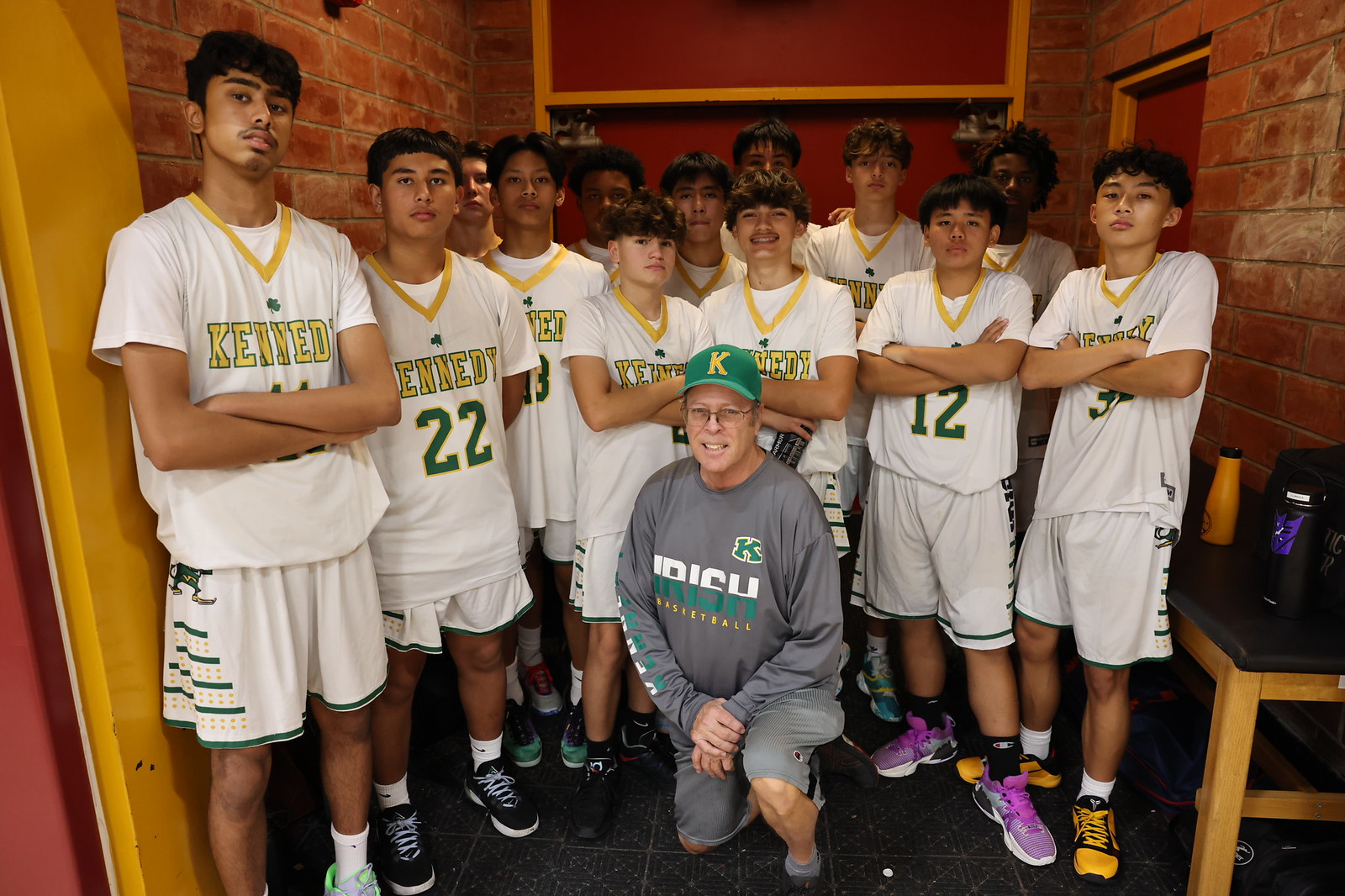In this image, we see a high school basketball team, likely from Kennedy High School, posing for a group photo. The players are dressed in matching white jerseys and shorts, featuring yellow and green numbers and letters, with "Kennedy" prominently displayed in yellow against a green border. Most of the boys have their arms folded, although a few have different postures. At the center of the group, the coach is kneeling down, wearing an all-gray outfit that includes shorts, socks, and a shirt which reads "Irish basketball." He also sports a green cap with a yellow "K" on it. This scene takes place in a room with red brick walls, partially visible red doors, and a red bulletin board nearby. To the right of the team, there is a wooden table with a black surface, an orange drink container, and a black coffee machine. The overall composition captures the spirit and unity of the team, ready for their next challenge.